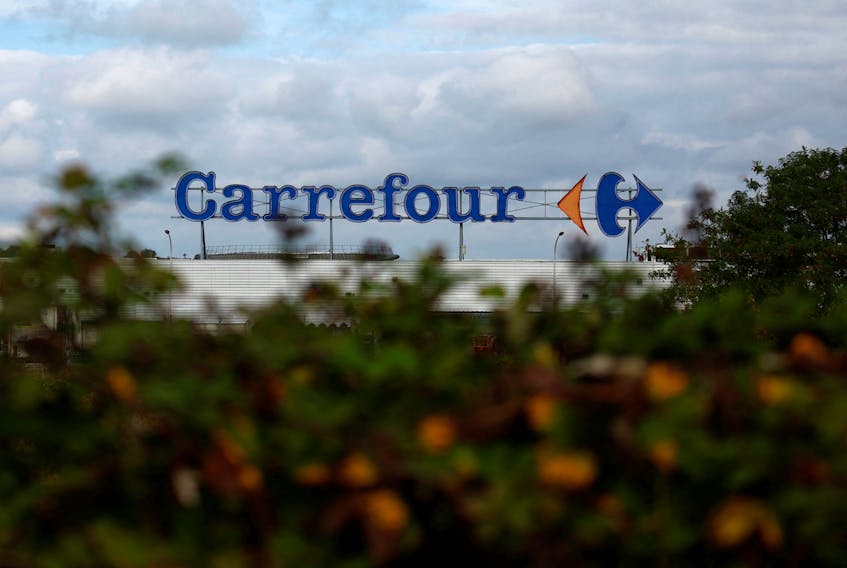In this photograph, the focal point is a prominently displayed sign atop a long, low, white building that stretches horizontally across the entire frame. The sign features the word "CARREFOUR" in bold blue letters, mounted on four support beams extending from the roof. To the right of the text, the logo comprises an orange triangle pointing left and a blue geometric shape pointing right. Above, the sky is heavily clouded with thick gray and white clouds, allowing only small patches of light blue to peek through. The foreground is dominated by a blurred hedge adorned with red berries or red fruits and some orange and green floral textures, adding a touch of color to the otherwise industrial scene.